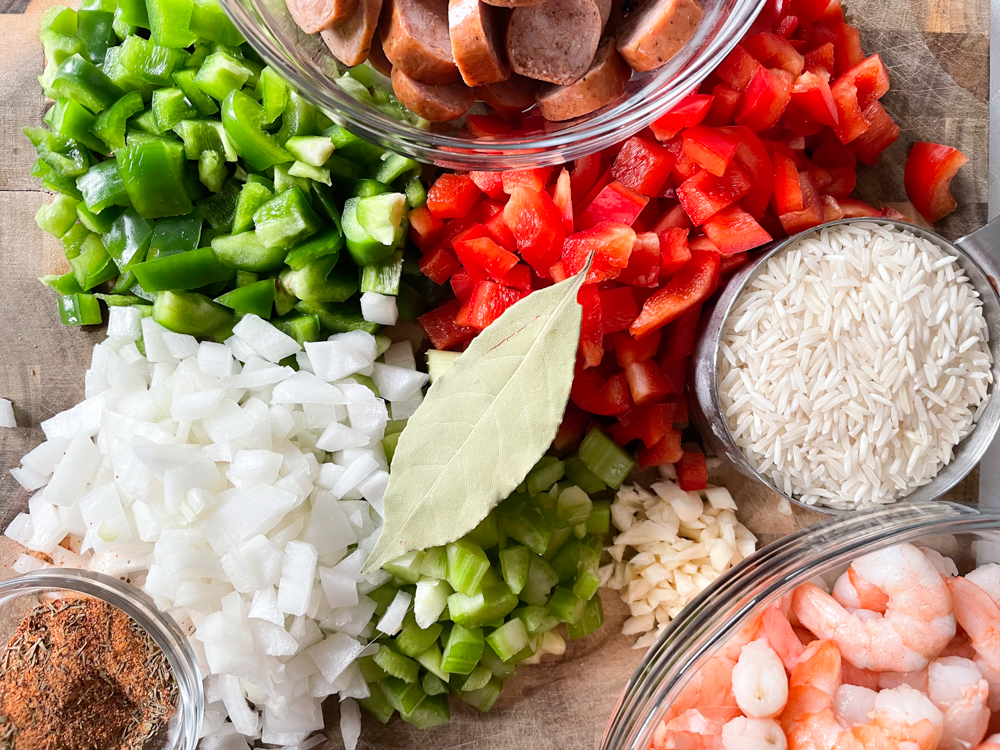This color photo, taken from a top-down perspective, showcases an array of ingredients meticulously arranged on a wooden cutting board, appearing prepped for an elaborate meal. Dominating the scene are four vibrant piles of chopped vegetables: green bell peppers, red bell peppers, white onions, and celery, all centered around a single bay leaf. To the right, a silver measuring cup holds a portion of white rice, while nearby, a small pile of minced garlic adds to the culinary mix. The lower right corner features a glass bowl brimming with fresh shrimp, contrasting with a large glass bowl at the top, filled with slices of Polish sausage. A small glass bowl of brown seasoning, possibly a cayenne pepper and herb mix, sits on the lower left. The vivid colors and neat arrangement suggest this could be a styled photograph suitable for a cooking magazine or advertisement, providing a feast for the eyes and an invitation to culinary creativity.